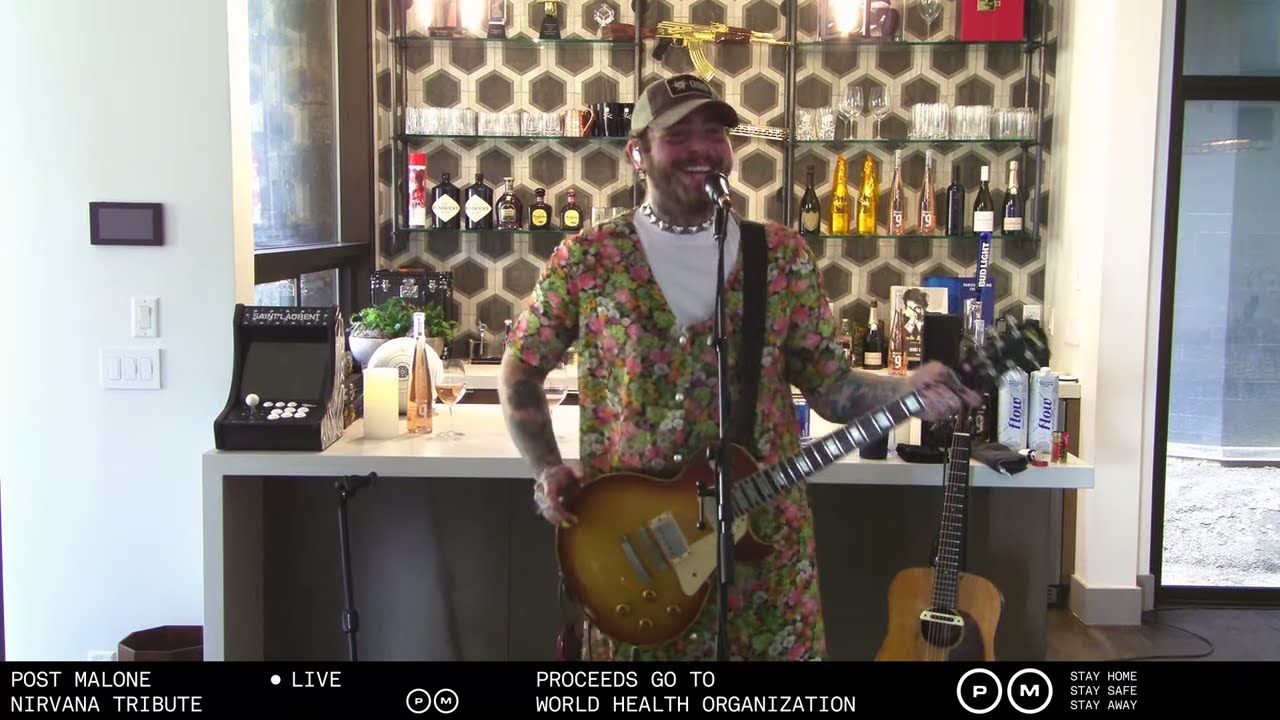In this vibrant and evocative photograph, Post Malone stands beaming with a broad smile, his face glowing with a bright reddish hue. He's dressed in a colorful ensemble, featuring a white t-shirt under a green, pink, and white romper, accessorized with a silver necklace and a rugged tan baseball cap. Post Malone is captured holding a tan electric guitar, positioned in front of a microphone. Behind him is a home bar setup filled with shelves and counters laden with an assortment of bottles, glasses, and a cash register. Another guitar is visible, propped up against the bar to his right. The bottom of the image bears the text: "Post Malone Nirvana Tribute Live. Proceeds go to the World Health Organization. Stay home. Stay safe." This visually rich moment encapsulates the buoyant spirit and charitable intent of the performance.